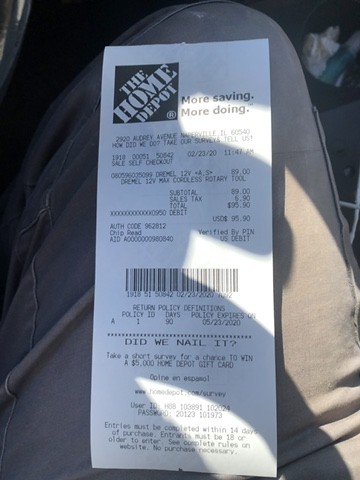This photograph captures a Home Depot receipt placed on a person's leg, clad in gray-colored pants, with the leg visible from thigh to knee. The receipt, printed on white paper, is partly illuminated by sunlight filtering in from the right, casting shadows and creating reflections, including the shadow of a hand across its surface. Crumpled paper objects are seen in the upper right-hand corner of the image. Prominently featuring the Home Depot logo and the slogan "More Saving, More Doing" at the top, the receipt lists the store's address as 2900 Audrey Avenue, Naperville, Illinois, 60540. It shows a total purchase amount of $95.90 charged to a debit card. Additionally, it includes details about a 90-day return policy expiring on May 23, 2020, and provides instructions for a customer survey that must be completed within 14 days of purchase, noting that entrants must be 18 or older. There is also a barcode and a section mentioning the survey, underscored by the phrase “How Did We Do? Take Our Survey and Tell Us.”